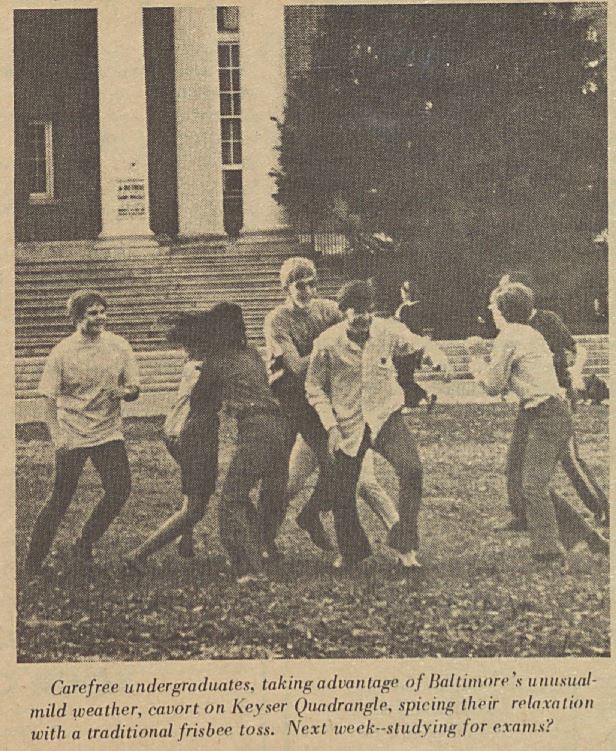This black and white photograph captures a lively scene on a university campus. In the background stands a grand building characterized by large white pillars and extensive staircases, leading up to a facade with sizable windows and a dark wall. To the right of the staircase, a massive tree adds to the serene atmosphere. In the foreground, a well-manicured garden or park area is visible, where students, both male and female, are energetically playing and socializing. The bottom of the image features a caption that reads: "Carefree undergraduates taking advantage of Baltimore's unusually mild weather, congregate on the quadrangle, spicing their relaxation with a traditional frisbee toss. Next week, studying for exams?"